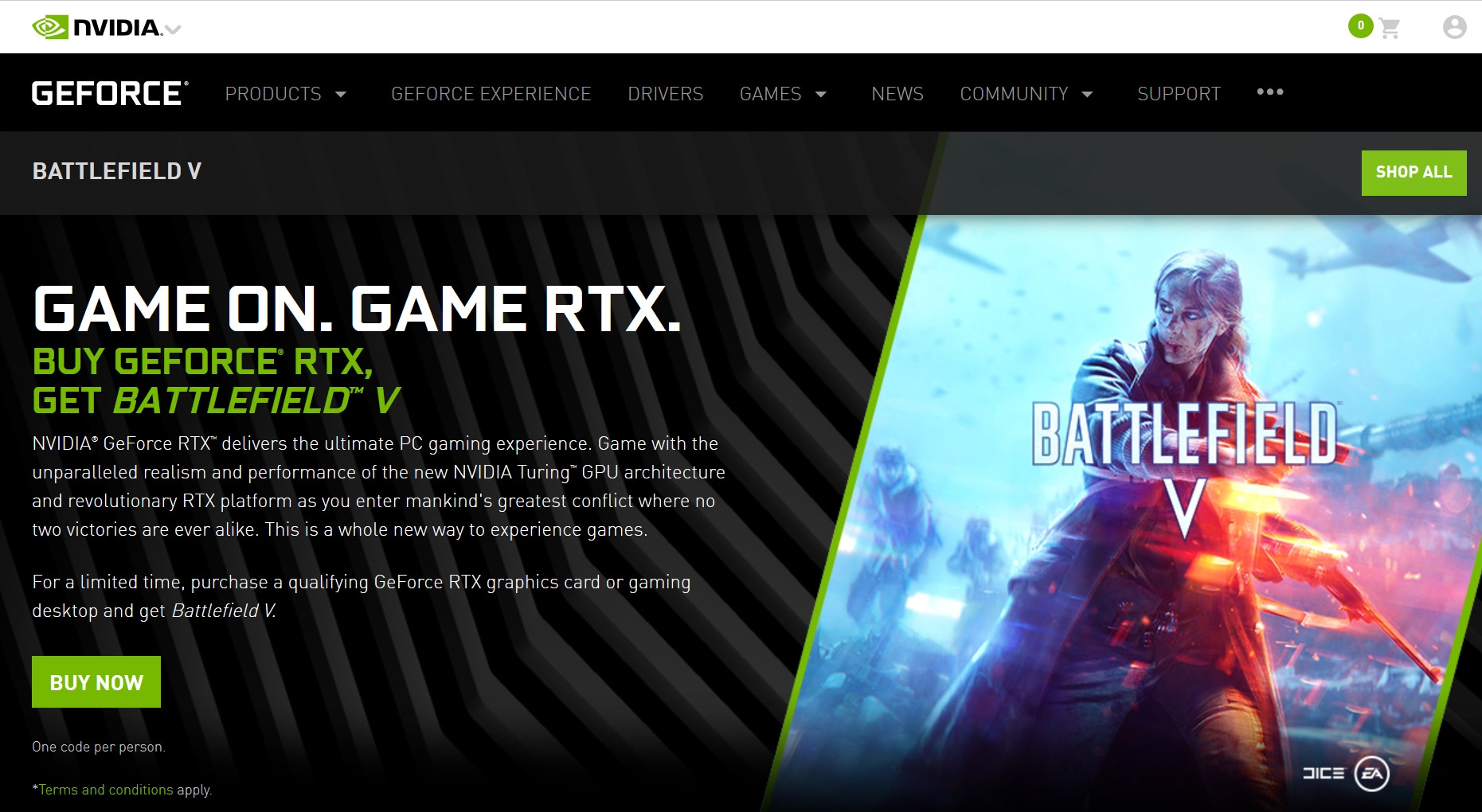The image features a prominently displayed white header at the top, emblazoned with the "NVIDIA" brand name accompanied by the company's iconic green logo. On the upper right corner of the header, there is a shopping cart icon and a profile picture symbol. Just below this, on the top left corner against a black background, the text "GeForce" is presented in white.

A toolbar is positioned beneath the "GeForce" label, offering a menu with several categories: "Product," "GeForce Experience," "Drivers," "Games," "News," "Community," and "Support." Further down, the text "Battlefield V" is displayed, with a green button labeled "Shop All" situated nearby.

The section below features the tagline "Game On, Game RTX, Buy GeForce RTX, Get Battlefield V." The accompanying description reads: "NVIDIA GeForce RTX delivers the ultimate PC gaming experience. Game with the unparalleled realism and performance of the new NVIDIA Turing GPU architecture and revolutionary RTX platform as you enter mankind's greatest conflict where no two victories are ever alike."